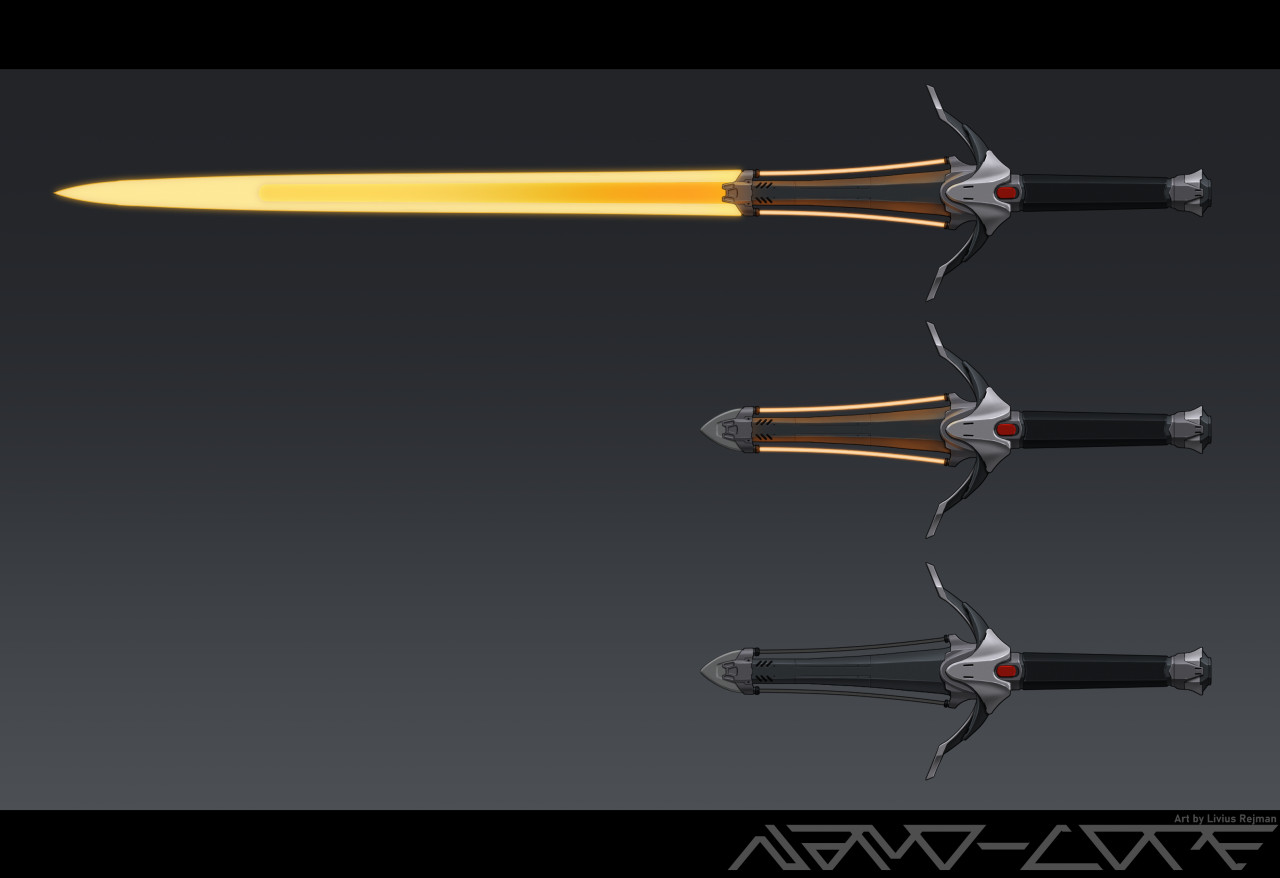The image is an animation drawing with hyper-realistic details, featuring three stylized swords or stilettos on a gradient background transitioning from dark gray to light gray. The composition is framed by black bars at the top and bottom; the bottom bar includes an inscription reading "Art by Livius Ryman," along with some undecipherable symbols.

The main focus of the image is the three swords depicted in different stages of illumination. The top sword is the most striking, extending almost the full width of the image. It features a vibrant yellow glowing blade with a darker orange core, giving it an almost ethereal appearance. The hilt and handle are black with metallic gray accents, including a red dot at the base of the hilt where the handle meets.

Below the top sword is a middle sword which retains the same black handle and gray hilt with the red dot, but only the hilt glows in brighter yellow with streaks of the same color extending slightly into the blade, which remains dark gray.

The bottom sword is the most subdued, showing a purely dark gray blade, with the same black handle and gray metallic hilt featuring the red dot, but without any glowing effects. The V-shaped hilt of each sword bends outward, highlighting their stylistic consistency. 

Overall, the image portrays the gradual activation of a sword, suggesting a transformation from a dormant state to a fully energized weapon, possibly portraying different stages of readiness or power.